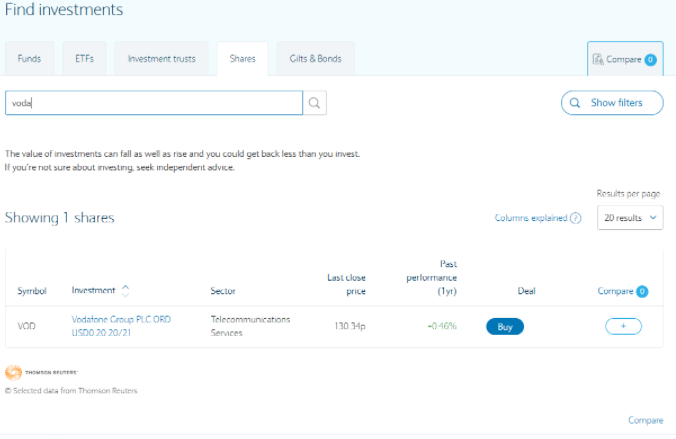The screenshot captures a website interface, likely viewed on a desktop or laptop, designed for financial purposes under the moniker "Fine Investments". At the top, a blue border prominently displays the website's name, "Fine Investments", accompanied by several navigation options, including "Funds", "ETFs", "Investment Trusts", "Shares", "GIFTS", and "Bonds". The "Shares" option stands out in white, indicating it is currently active, while the others are grayed out.

Beneath the navigation bar, on the left side, a search box appears with the partially typed text "V-O-D-A", suggesting a search query in progress. To the right of the search box, there's a button labeled "Show Filters" for refining search results.

The main content area, set against a white background, contains text addressing the value of investments. The visible data outlines the details for one specific share, including its symbol, investment sector, last closed price, past performance, and options for dealing and comparison. A button labeled "Compare" is available below this section.

The layout is intuitive, placing essential tools and information within easy reach, enhancing user experience for those managing and comparing investments.